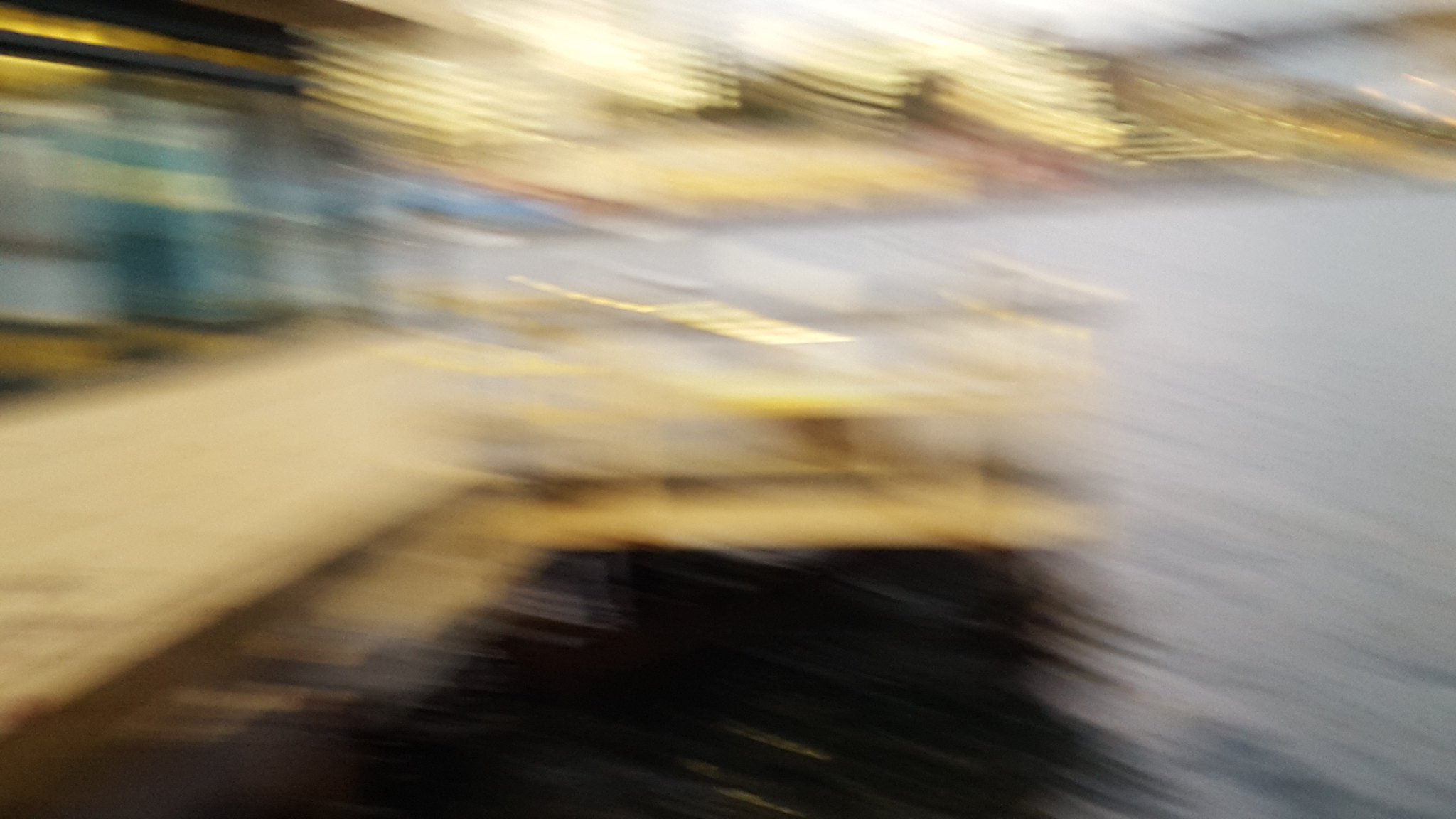This photo, though captured with significant motion blur, depicts a scene by a large body of still water that appears to be a lake, indicated by its almost black dark bluish-gray color. On the left side, there is a light brown or beige-colored dock with a small wooden pier extending over the water. Adjacent to this, there's a light gray road or sidewalk, possibly accompanied by a building whose features remain indistinguishable due to the blur. In the background, faint lights suggest distant buildings or another dock. The overall scene is dark, possibly taken near dusk, enhancing the obscure and shadowy atmosphere.